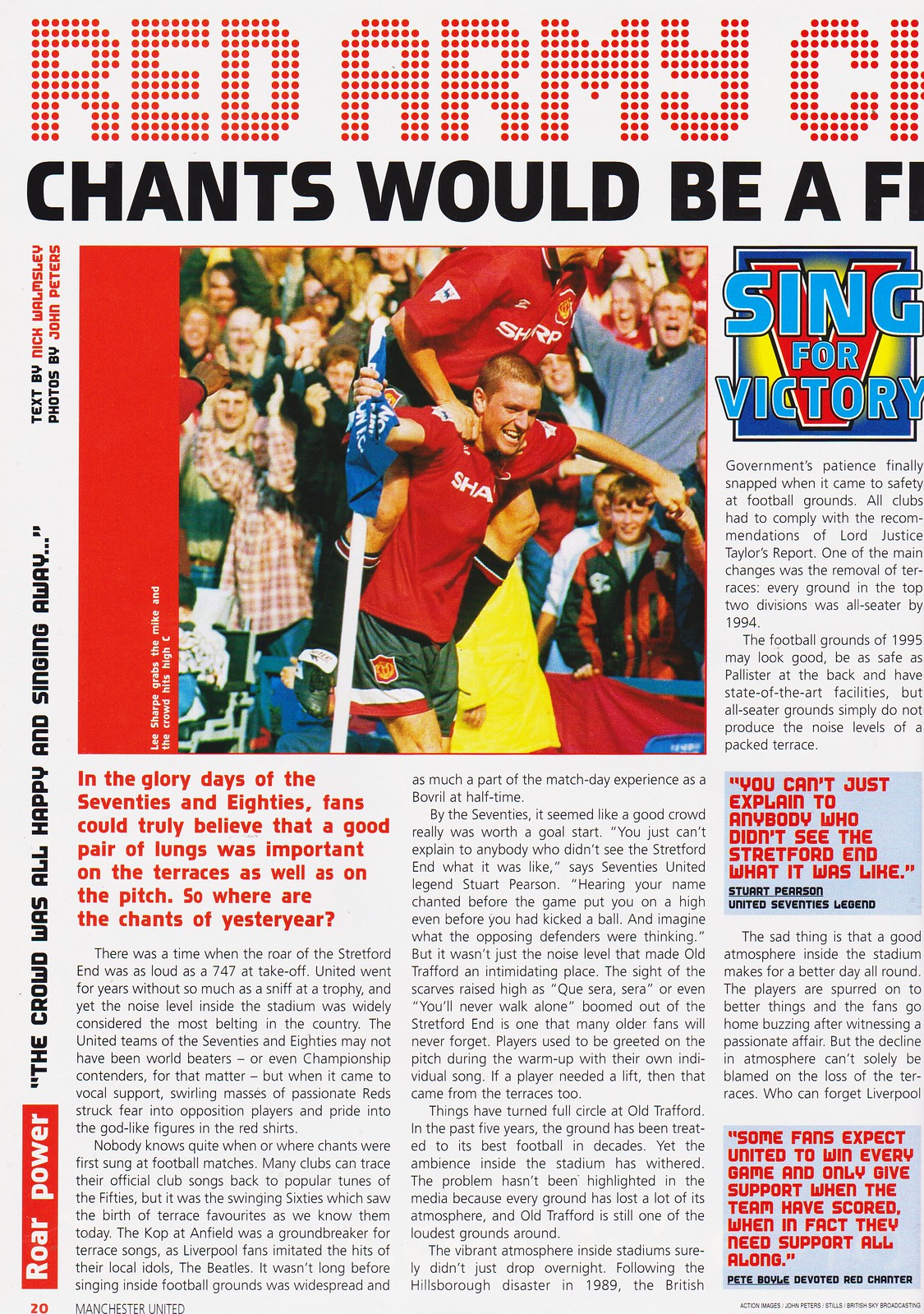This image is a page taken from a sports magazine, likely centered around soccer. The background of the page is a solid light gray or white, and it's immediately clear that the design spans across two pages, as the top text reads, "Red Army," followed by truncated words due to the page cut-off. The partial headline hints at the phrase "Chance would be a..." but it's incomplete. Below this, a large photograph captures two soccer players in red jerseys with white text and dark shorts celebrating a victory; one player is on the other's shoulders. Behind them, there’s a jubilant crowd. Text beneath the photo nostalgically reflects on the glory days of the 70s and 80s, emphasizing the importance of vocal support from the terraces. Notable colors in the image include red, black, blue, yellow, dark blue, green, and tan. The photograph occupies the top center, while most of the accompanying text is positioned towards the bottom and right side. Additional graphics are present, with "roar power" along the left edge and "sing for victory" in the third column on the right.